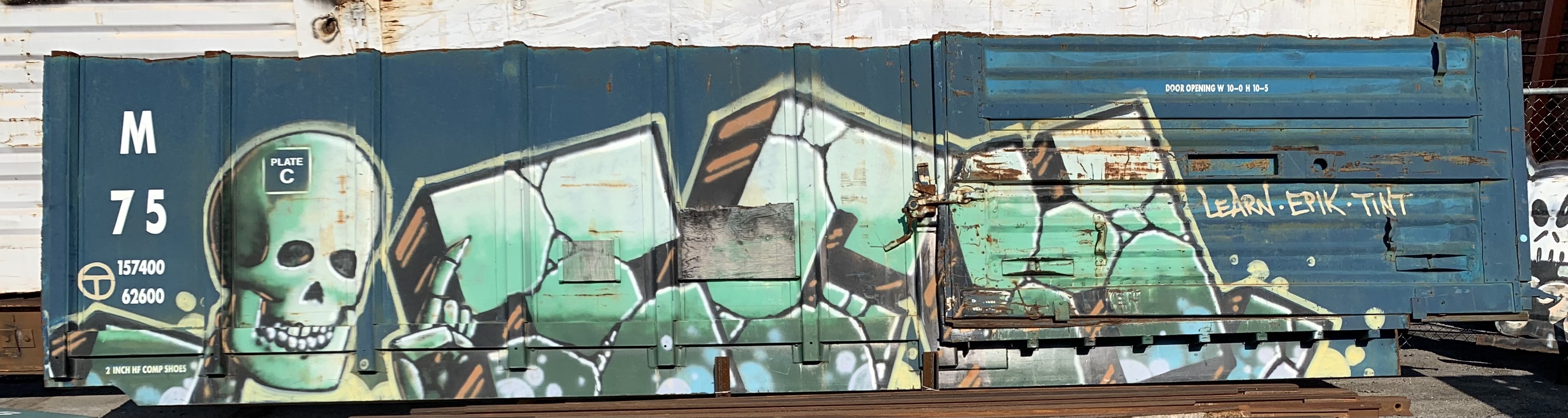The image shows a large, dark blue metal shipping container or train car, appearing somewhat rusted in areas and set against a white wall. The container is covered in intricate graffiti, predominantly using teal and white colors with black and orange shading. On the left side, there's a giant, stylized light blue skull, complete with visible teeth and eye sockets, which extends a hand with a pointing finger towards the center of the container. Near the skull, the number "75" along with the letter "M" is prominently displayed, likely indicating original container markings. To the right of the skull, three cracked, cubical blocks resembling rocky letters sit in a somewhat collapsed arrangement. Further right, are the bold uppercase letters spelling "LEARN EPIC TENT." At the very edge of the right side of the container, there's a visible chain-link fence and what appears to be a painted face on another metal section, possibly part of the container or nearby structure. The container rests on a brown metal support that runs underneath it.